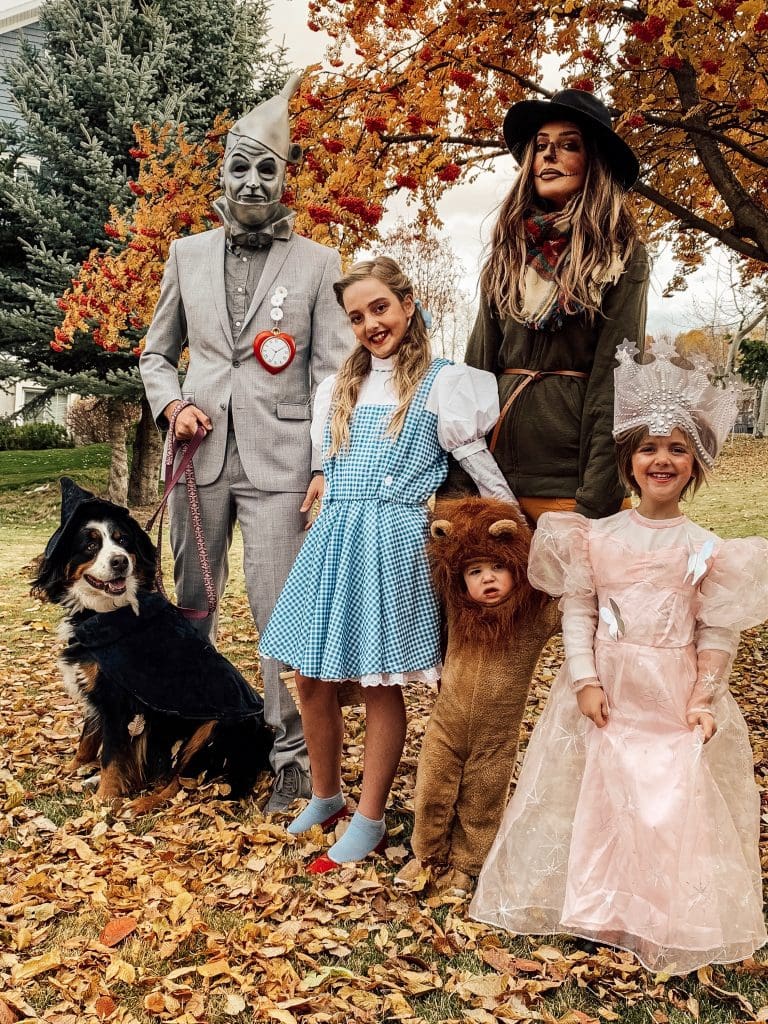In this outdoor, daytime photograph set in the colorful season of fall, a family of five and their dog are posing in a large, green yard strewn with yellow and brown dead leaves. The backdrop features a mix of trees adorned with vibrant orange, red, and yellow leaves, along with one green pine tree. Starting from the left, the man is dressed in a detailed Tin Man costume with a gray suit, matching gray makeup, and an oil can funnel hat. He is holding the leash of a black and white dog wearing a whimsical witch's hat. Next to him, a young girl stands out as Dorothy from the Wizard of Oz, donning a blue and white dress, her hair styled in pigtails, and traditional blue socks paired with red slippers. Beside Dorothy, a small child is costumed as a lion, fitting snugly in a one-piece outfit. To the right, another little girl is capturing the role of Glinda the Good Witch, adorned in a frilly pink dress with silver butterfly embellishments and a large crown. In the back, the mother rounds out the Wizard of Oz theme as a scarecrow, complete with a wide-brimmed black hat. The overall setting, with its rich autumnal hues and the family's coordinated costumes, evokes a festive and heartwarming scene.